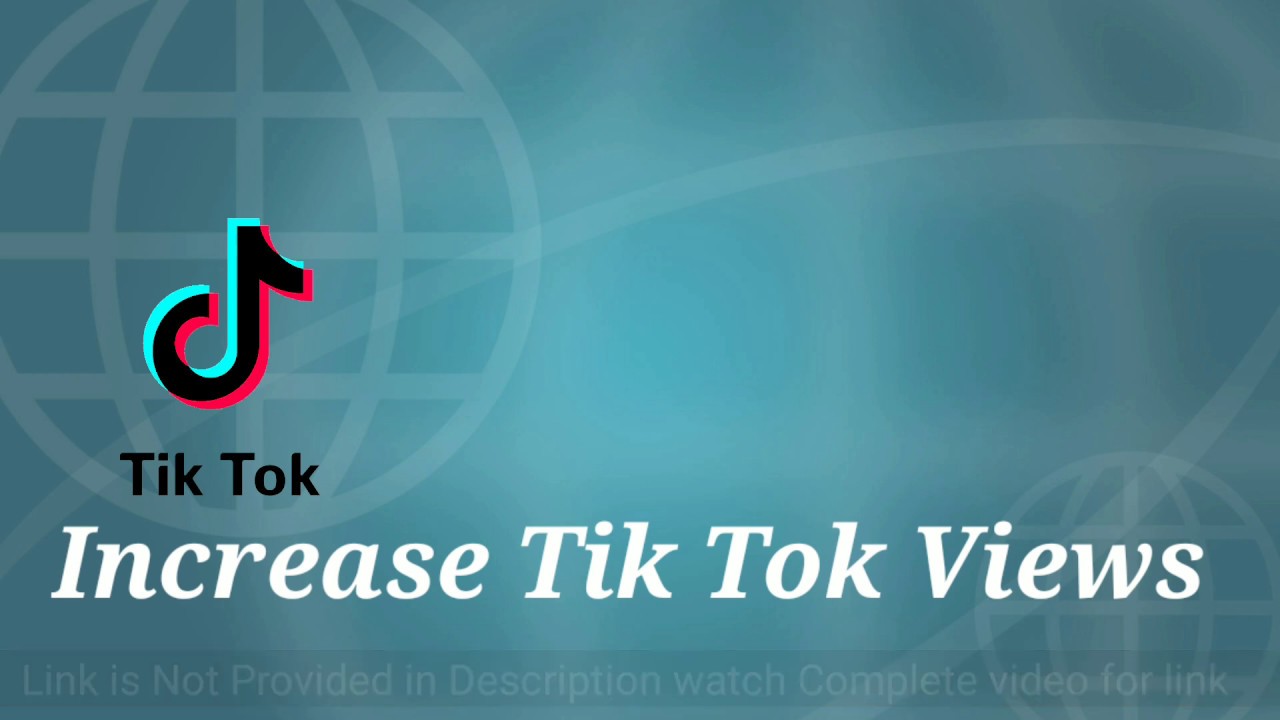A horizontally oriented screenshot appears to be related to TikTok. Centered in the image is the recognizable TikTok icon, featuring a black music note with red and light blue accents on either side. Directly beneath the icon, the text "Tik Tok" is displayed, unusually separated into two words in black ink. Below this, the italicized phrase "Increase TikTok views" is written in white lettering.

The background of the image has a grayish-green hue, with a faint graphic of a globe, adding a sense of global connectivity. At the bottom, there is a somewhat inconsistent text in grayed-out font stating, "LINK IS NOT PROVIDED IN THE DESCRIPTION. WATCH COMPLETE VIDEO FOR LINK," with some words unusually capitalized.

The format and context suggest that this screenshot might be from a platform other than TikTok, possibly a YouTube video or an online tutorial, as indicated by the non-standard presentation of the "Tik Tok" text.